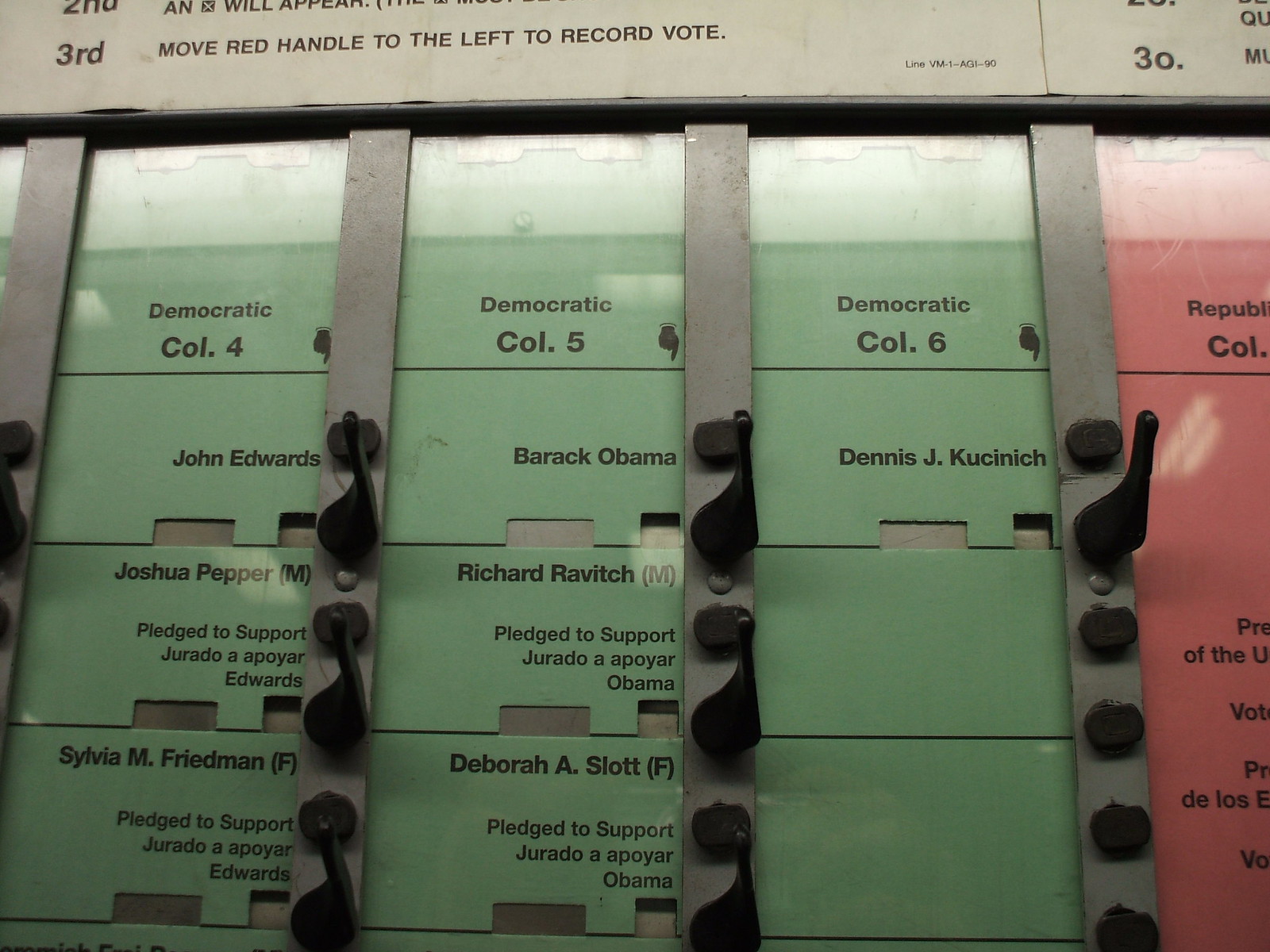This is a color photograph depicting the interior of a voting machine. The machine features four vertical columns with metal bars and knobs. The first three columns on the left side are green with black text printed on them and are labeled "Democratic." They correspond to the designations COL4, COL5, and COL6. These columns list candidates including John Edwards, Joshua Pepper, Sylvia Friedman, Barack Obama, Richard Rabovich, Deborah A. Slott, and Dennis Kucinich. The far-right column is red, marked "Republican," though the text is mostly unreadable.

Inside the voting machine, the candidates' names are arranged behind glass, with little black dots and tabs next to each name. The instruction on a notice in the booth indicates to "move red handle to the left to record vote," adding a critical detail for voters. The setting inside the booth appears somewhat dimly lit, enhancing the visibility of the colored columns and the contrasting black text.